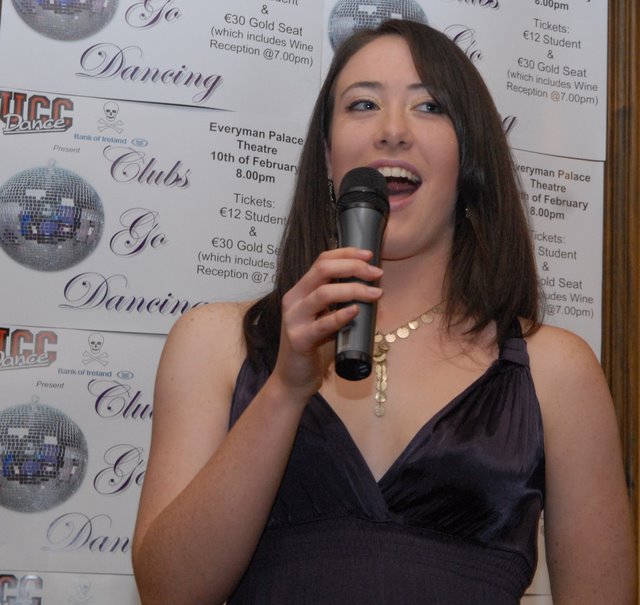This photo captures a joyful young woman in her early 20s, dressed in a stylish low-cut, sleeveless black cocktail dress. Her shoulder-length brown hair frames her face as she holds a microphone close to her mouth, wide open in laughter or mid-speech. A striking gold necklace with metal-like circles cascading down to her neckline adds a touch of elegance to her ensemble. Behind her, the wall is plastered with multiple posters advertising a dance event at the Everyman Palace Theatre on the 10th of February at 8 p.m., with ticket prices listed as €12 for students and €30 for gold seating, the latter including a wine reception at 7 p.m. The repeating graphics and text on the posters—featuring phrases like "UCC Dance," "Clubs Go Dancing," and an image of a disco ball—create a lively backdrop that contrasts with her spirited expression and poised presence, suggesting she's either performing or addressing the audience at this event.